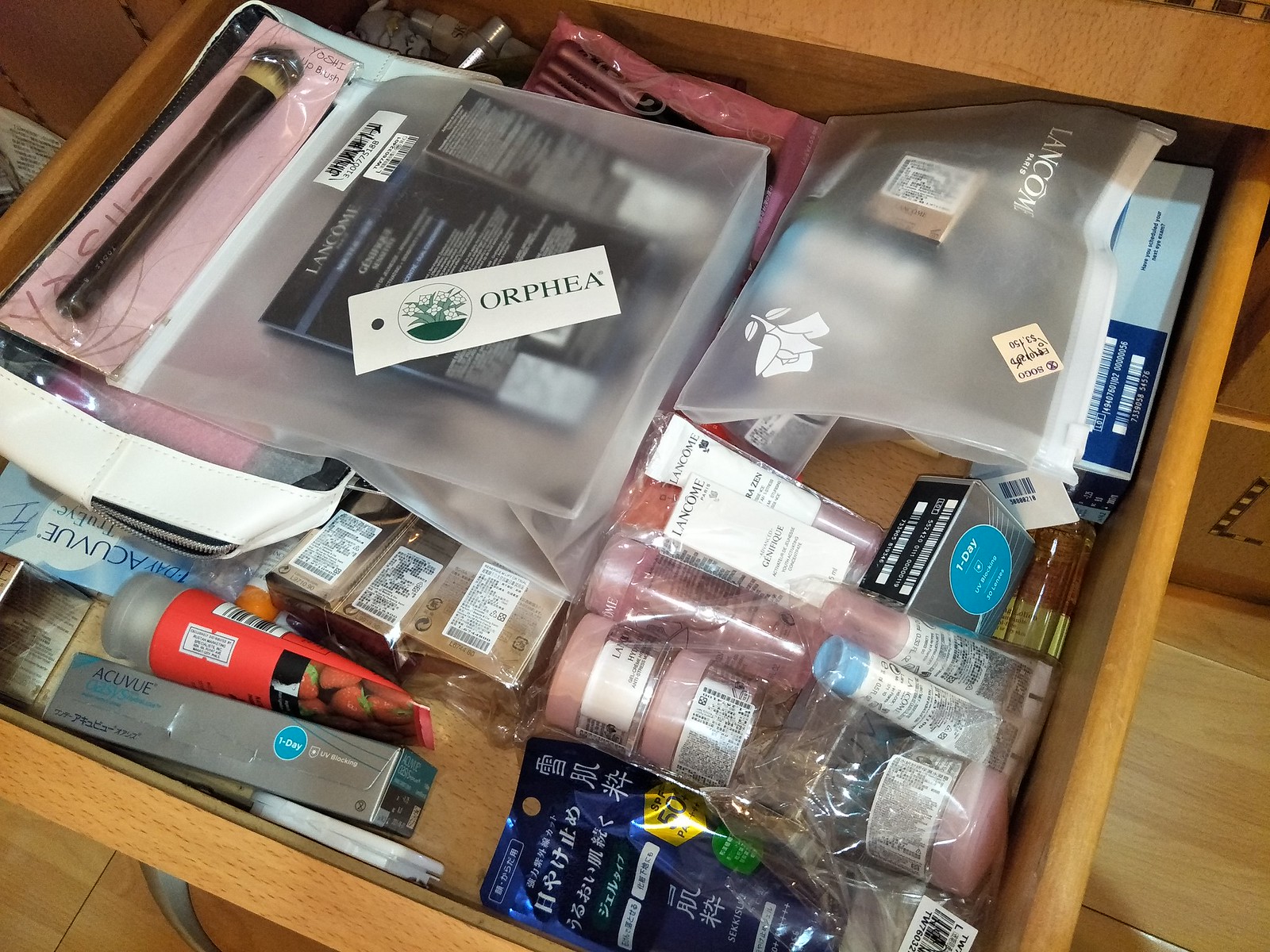A highly detailed color photograph captures a close-up view of an open drawer filled with various cosmetic products. Due to the proximity of the camera, it is challenging to determine whether the drawer is part of a desk or a kitchen counter. Inside, a diverse array of items is visible, with some products displaying labels in an unidentified Asian language. Notably, several products are branded with the Lancôme label, indicating that this might be a dresser drawer containing cosmetics.

The contents within the drawer include six to ten small containers resembling eye cream pots, along with a variety of other cosmetic items. Among the assortment, there are a few makeup brushes and zip bags, one of which is labeled with the name "Sophia." Additionally, there are products from One Day Acuvue, suggesting the presence of contact lens-related items within the drawer.

The drawer appears organized yet densely packed with several dozen cosmetic and related products. The detailed close-up provides a glimpse into a well-stocked cosmetic collection, featuring both Western and Asian beauty products.